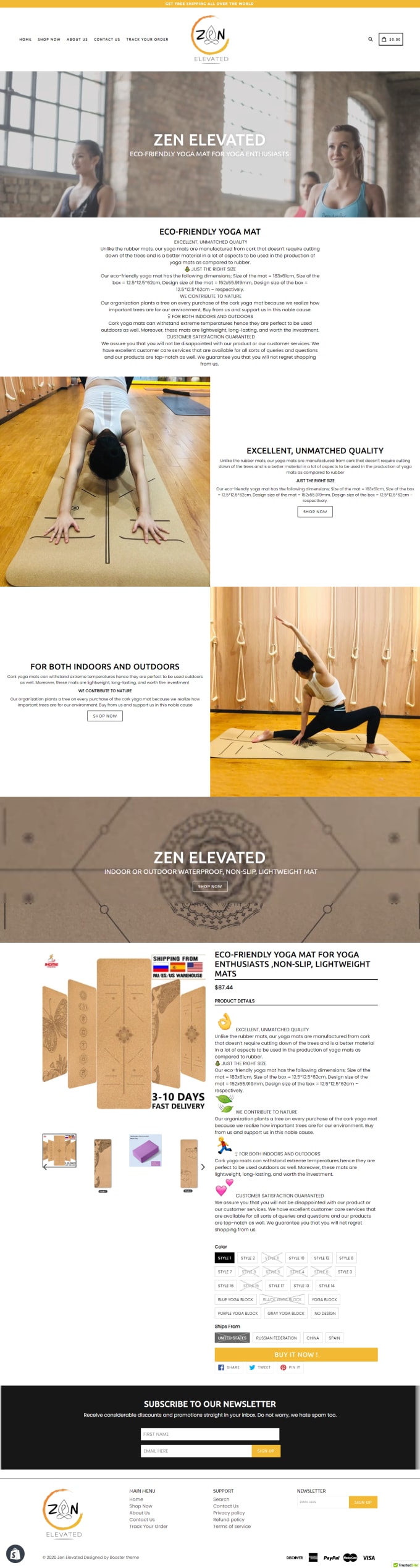This well-crafted advertisement captures the essence of the "Zen Elevated" product line. The website header is highlighted by a striking orange stripe that runs prominently across the top. At the center of this stripe is a circle emblem featuring the word "Zen" in bold typography. Just below this, the central image presents the phrase "Zen Elevated" in crisp white letters, setting the tone for the sophisticated branding. A description follows beneath this primary image, though the details remain indistinct. Moving further down, the advertisement showcases a serene visual of a person positioned on a mat, poised on their hands and knees, embodying the tranquil state associated with being "Zen Elevated." Below this peaceful scene, there are images of brown boxes or envelopes, hinting at packaging or storage elements related to the product. Finally, an additional letter appears at the bottom right, though the content remains elusive due to clarity issues in the photo. Overall, the advertisement artfully combines elements of calm and organization, inviting viewers to explore the Zen Elevated experience.